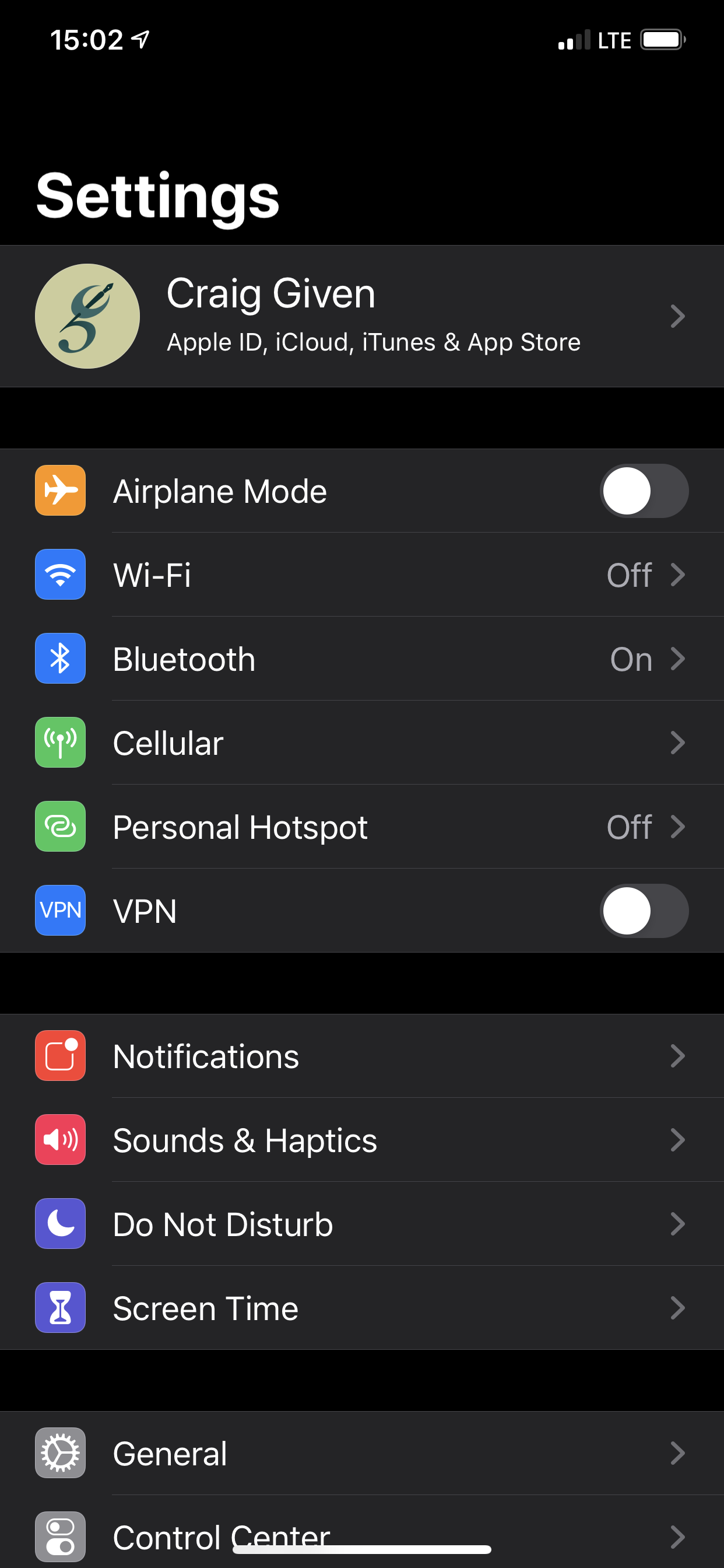This is a descriptive caption of a mobile phone screen capture in dark mode, showcasing the settings screen of an Apple iPhone. 

In the upper left corner, the time is displayed in military format as 15:02, adjacent to a navigation icon. Moving across the top edge to the right corner, there is a signal strength indicator showing two active bars, followed by the text 'LTE' in uppercase, and a nearly fully charged white battery icon.

Below, occupying the uppermost section of the settings interface, is a circular avatar indicating the phone owner's identity as Craig Given, with the text "Apple ID, iCloud, iTunes, and App Store" right underneath. This confirms that the device is an iPhone.

The central portion of the screen consists of various settings categories, each delineated with corresponding toggle options or chevrons for extended configurations. These include:
- Airplane Mode (toggle option)
- Wi-Fi (off option)
- Bluetooth (on/off option)
- Cellular (chevron for more options)
- Personal Hotspot (on/off option)
- VPN (toggle option)
- Notifications (chevron for more info)
- Sounds & Haptics (chevron for more info)
- Do Not Disturb (chevron for more info)
- Screen Time (chevron for more info)

The lower portion visible in the screenshot lists 'General' and 'Control Center,' both with right-facing chevrons indicating further submenus.

The detailed layout and icons all reinforce that this is indeed an iPhone settings menu in dark mode.